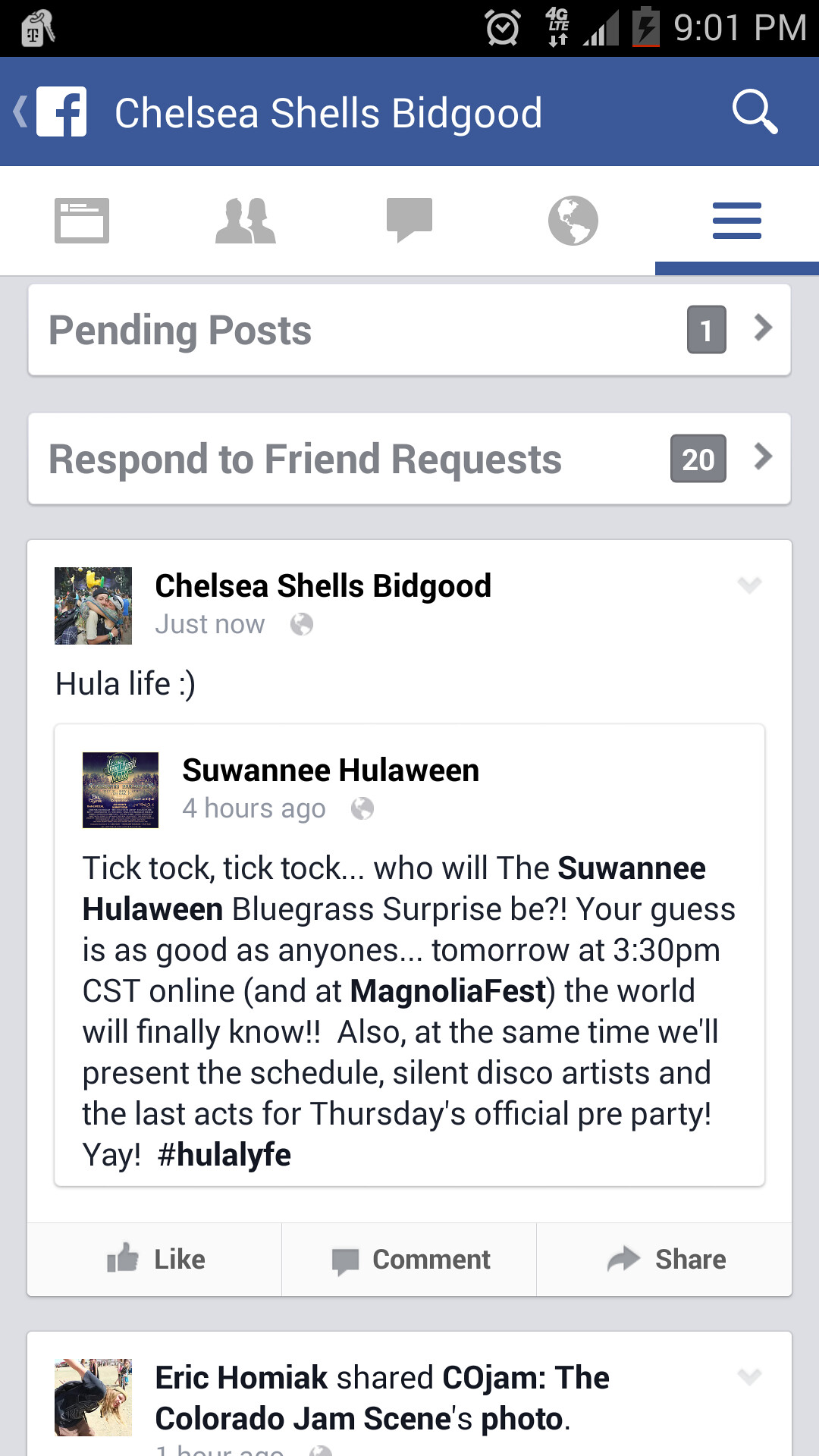This image is a screenshot of a cell phone displaying a Facebook post. At the top of the screen, the status bar shows it is 9:01 p.m., with a low battery, 4G signal strength, and an alarm clock symbol. The Facebook app interface is prominent, with the classic blue heading featuring a Facebook logo and a search bar symbol, and a hamburger menu icon. The profile name "Chelsea Shells BidGood" is identified twice in the header.

The main content of the image is a post from Chelsea Shells BidGood, which reads "Hula Life ✨." Just below this, there is a response from "Suwannee Hulaween" posted four hours ago, stating: "Tick-tock, tick-tock! Who will the Suwannee Hulaween bluegrass surprise be? Your guess is as good as anyone's! Tomorrow at 3:30 p.m. CST online and at Magnolia Fest, the world will finally know. Also at the same time, we'll present the schedule, silent disco artists, and the last acts for Thursday's official pre-party. Yay! #HULALIFE." At the bottom of the post are options to Like, Comment, and Share, and there's a note "Eric Homeyaks shared Co-Jam: The Colorado Jam Scene’s photo."